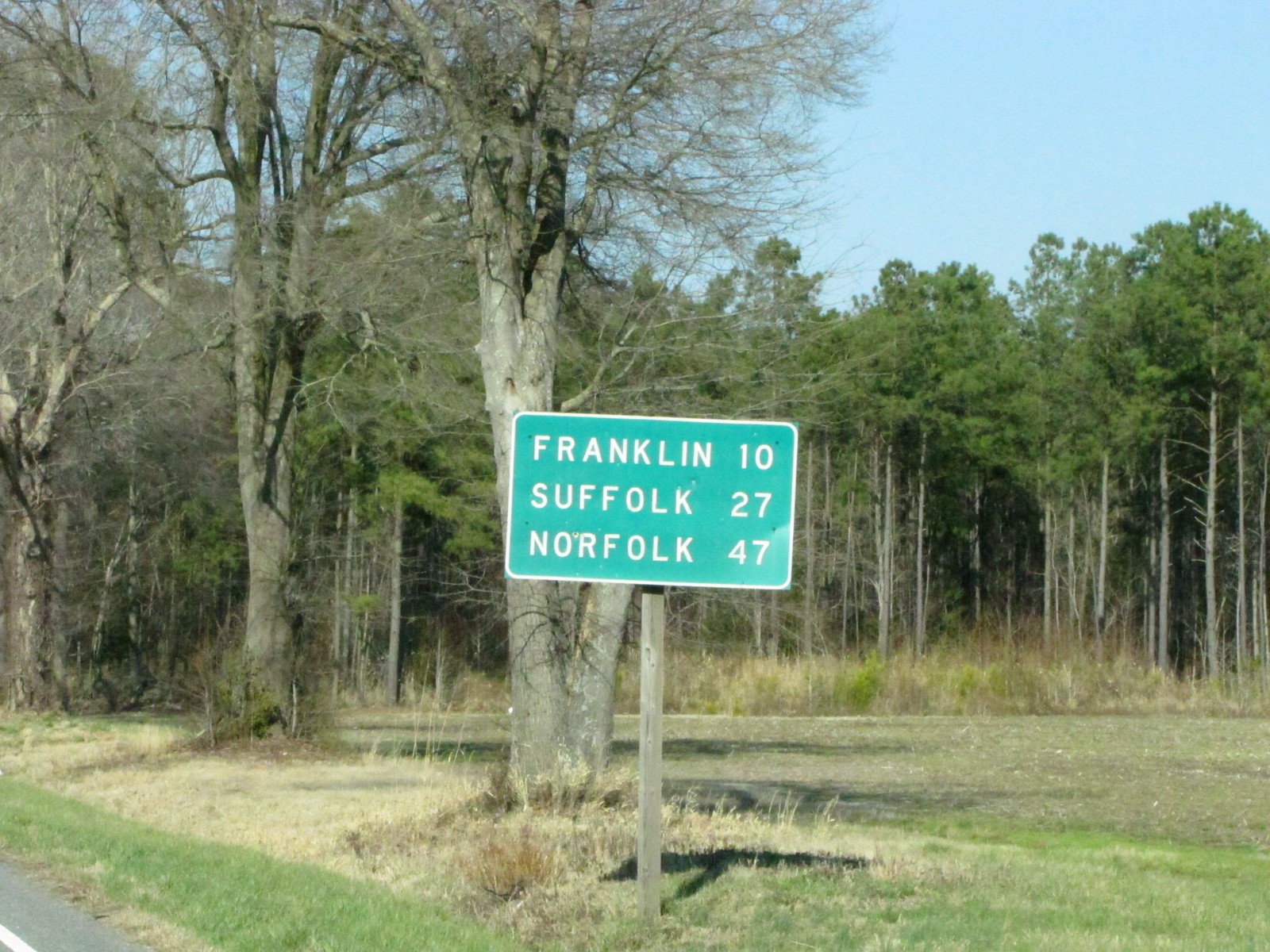This image, seemingly captured from a moving vehicle, showcases a vibrant yet varied landscape featuring a mix of brown and lush green grass in the foreground. A wooden pole supports a green rectangular mile marker sign with a white border. The sign displays three locations: Franklin (10 miles), Suffolk (27 miles), and Norfolk (47 miles) in bold white block letters. To the right of the sign, the ground casts a clear shadow, adding depth to the scene. The background is dominated by a dense grouping of trees, suggesting the presence of a nearby forest or woodland area. In the bottom right corner, a portion of the road and a distinct white line are visible, hinting at the perspective from within the vehicle.